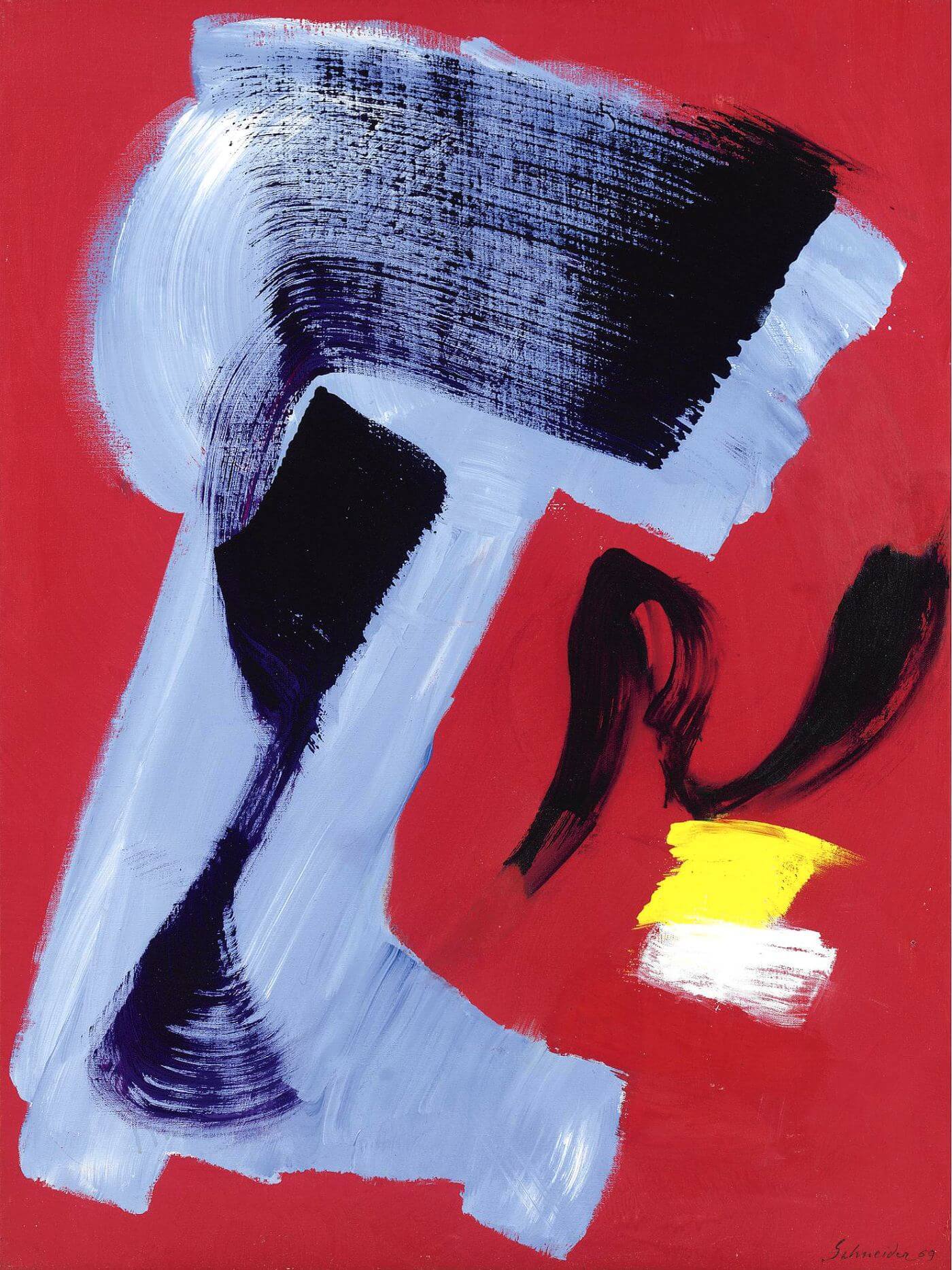The artwork is an abstract oil painting centered on a red background. Dominating the composition are expressive brushstrokes starting in the bottom left with sweeping motions of light blue paint that swirl upwards to the left before curving back to the right. Layered over the light blue are prominent black strokes that grow more solid as they ascend, intersecting and sweeping left before looping up and veering right again. These strokes create a sense of movement and depth, at points blending into a faint purple where they converge.

To the right of this central feature, additional brushstrokes add complexity. A striking black stroke begins by moving straight up before curving to the right and descending to connect with a yellow patch, and then rising again. Nearby, a patch of white paint and another of yellow paint are spread horizontally, adding contrasting highlights to the piece.

In the very bottom right-hand corner, a small signature in black letters, possibly accompanied by a date, marks the artist’s identity, though it is indecipherable. This distinctive abstract piece exudes an energetic and dynamic quality, with layered colors and intricate brushwork that might suggest a human form or simply evoke a sense of organized chaos. The painting is likely featured on an art website, possibly for sale, showcasing the artist’s striking use of color and form.